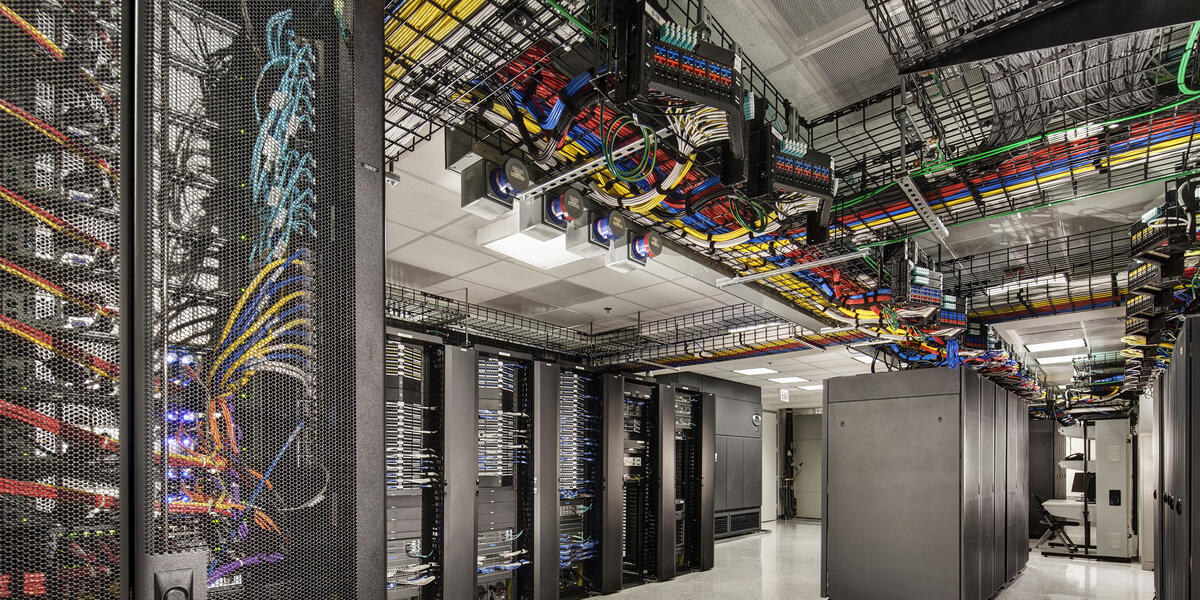The photograph depicts the interior of a technology building, specifically a server room or data center, characterized by its landscape layout. The room is filled with numerous large, black server cabinets positioned on a smooth, shiny grey laminate floor. The regular height ceilings are white with grey tiles, and feature extensive runs of multicolored wires—yellow, blue, red, green, and some orange—neatly organized within a black cage-like framework. These wires, which are clearly visible just below the ceiling, snake across the room and connect to the servers, particularly noticeable on the left side of the image where they enter the nearest set of cabinets. The space is well-lit with fluorescent lighting, highlighting the meticulous setup of the infrastructure. This detailed arrangement suggests the room is a high-capacity data center containing hundreds of servers, possibly housing data for an internet company.